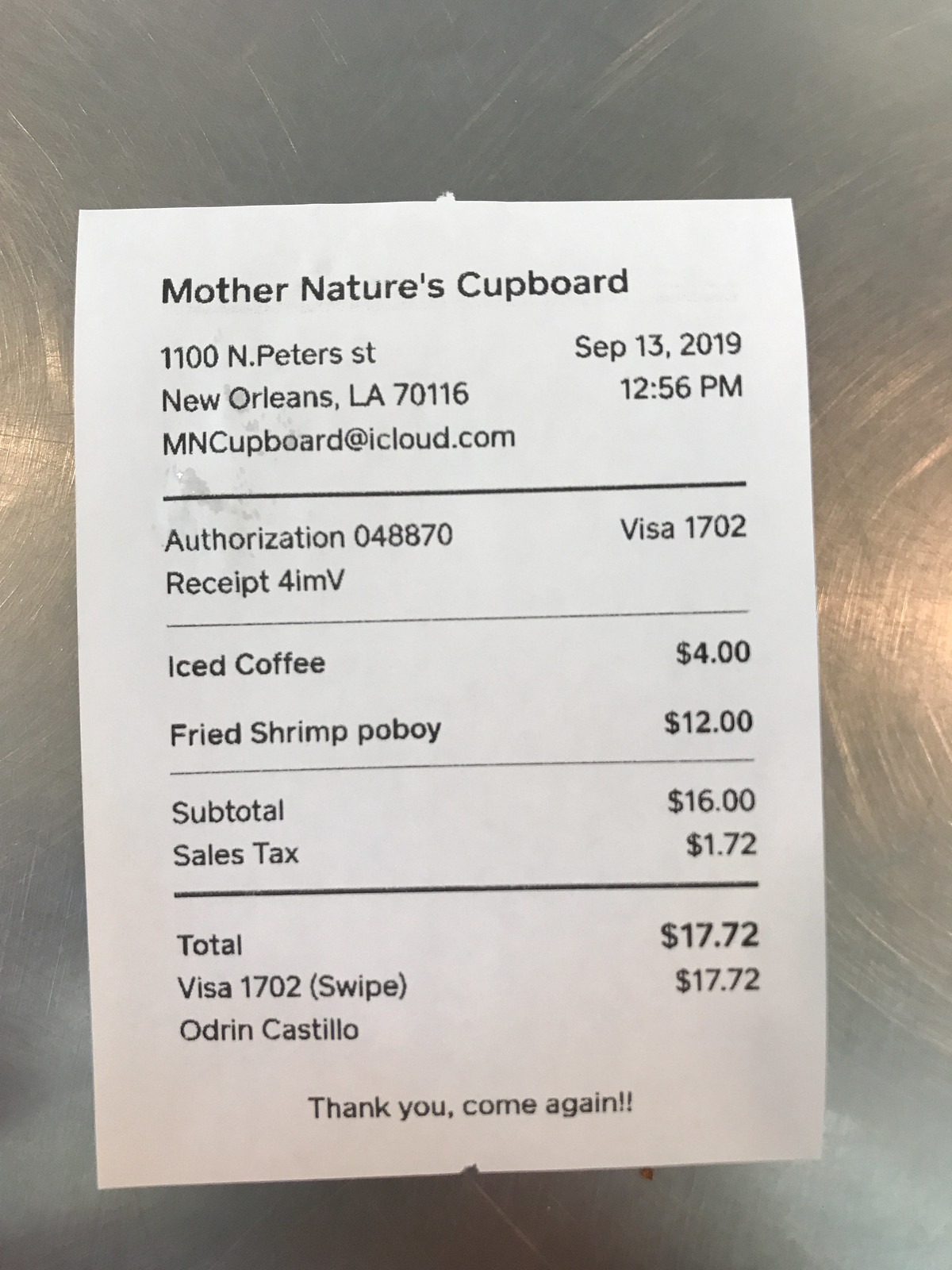A vibrant, high-resolution photograph captures a receipt resting on a meticulously brushed stainless steel surface likely belonging to an upscale kitchen or modern café setting. Subtle brush marks are visible on the metallic surface, adding texture and reflective qualities to the image. The receipt itself is relatively short, bearing the header "Mother Nature's Cupboard" with the accompanying address, "1100 North Peters Street, New Orleans, Louisiana, 70116" and contact email "MnCupboard at iCloud.com."

Dated September 13th, 2019 at 12:56 p.m., the receipt shows an authorization code "048870" and receipt number "4IMB." Payment was made via a Visa card ending in 1702. The itemized breakdown lists an iced coffee priced at $4.00 and a fried shrimp Po'Boy at $12.00, culminating in a subtotal of $16.00. With the inclusion of a $1.72 sales tax, the total amounts to $17.72, which matches the amount processed by Visa.

The bottom of the receipt is signed off with the name "Odren Castillo" and a friendly closing remark, "Thank you. Come again." The detailed presentation of the receipt, set against the clean and reflective stainless steel, lends an intimate glimpse into the moment of a simple yet satisfying transaction.